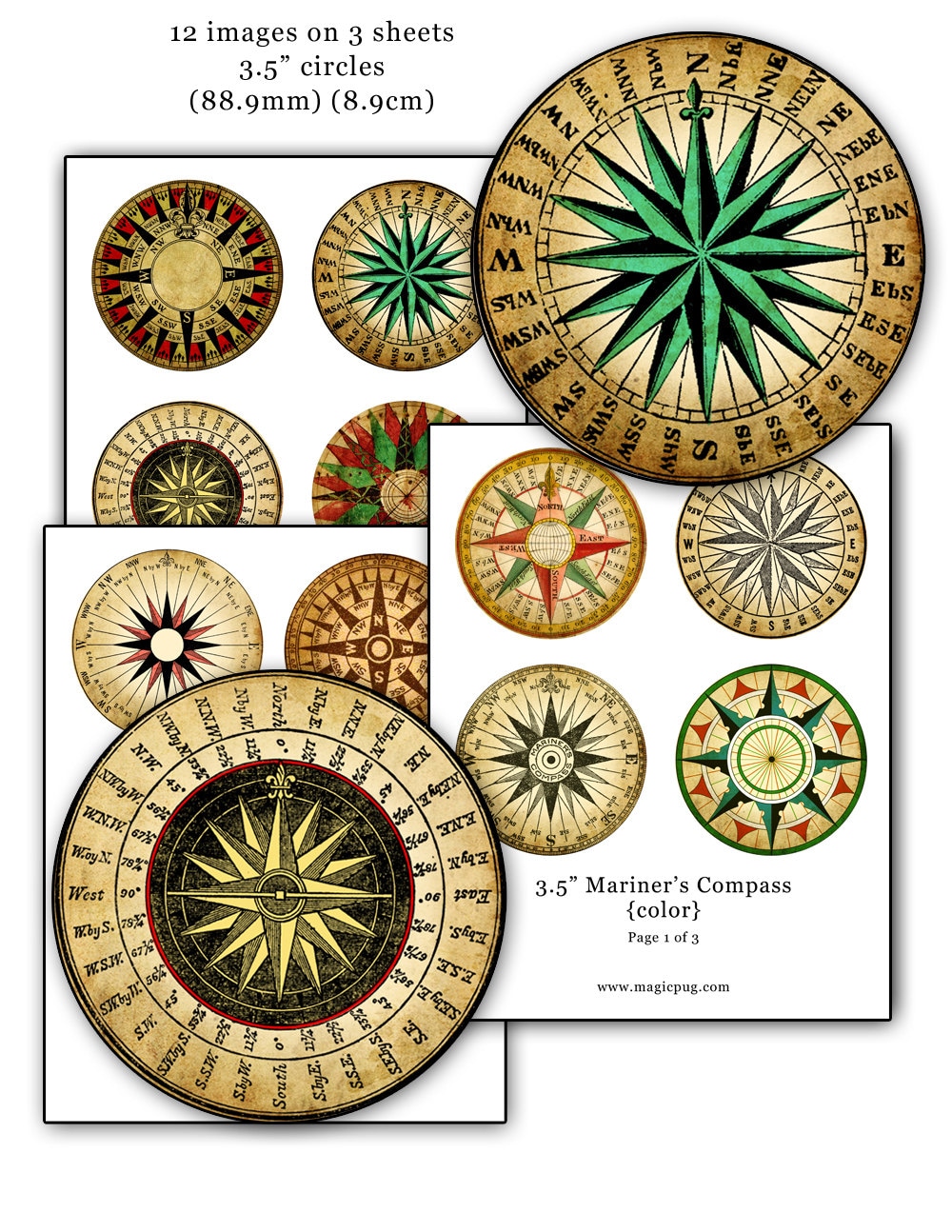The image depicts a detailed collage of various computer-generated Mariner's compasses in different colors and styles on three overlapping pieces of white paper. Each piece contains four distinct compass designs, totaling 12 images presented in 3.5-inch circles, equivalent to 88.9 millimeters or 8.9 centimeters. The compasses vary significantly in their markings and indicators, showcasing a range of designs that include intricate, spiky flower-like patterns. One piece of paper distinctly reads "3.5-inch Mariner's Compass" and illustrates the traditional directional indicators (e.g., North, West, Northeast). At the top of the image, text specifies "12 images on three sheets, 3.5 inch circles," while the bottom right includes a note that reads "3.5 inch Mariner's compass color, page one of three," along with a website URL: www.magicpug.com. Additionally, two enlarged designs from these pages are highlighted individually, one featuring a green spiky flower-like center in the upper right corner and another with layered black, white, or gray and beige tones in the bottom left. This detailed representation emphasizes the diverse visual styles and formats of the compasses.